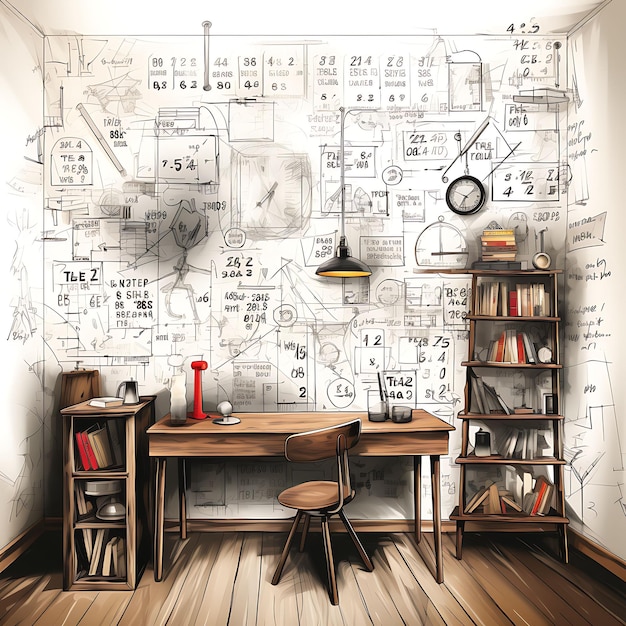This detailed digital drawing depicts an eclectic and busy end of a room styled as a scientist’s workspace. Central to the scene is a brown desk with a small chair, positioned beneath a black, dome-shaped hanging lamp that has a yellow interior. The desk holds a collection of objects, including oblong items—one distinctly red—and a jar with a paintbrush in it. Adjacent to the desk, to the left side, stands a taller bookcase with five wooden shelves filled with books and a coffee pot on top. To the right, there is a shorter bookcase of similar material, supporting additional books and various items.

The back wall is a canvas of creative chaos; it's predominantly cream-colored but covered with numerous hand-drawn sketches, numbers, letters, and schematic drawings, giving the impression that the wall itself has been used in place of traditional paper for brainstorming and jotting down ideas. At the center of this mural-like wall, there is a black clock with a white face and clear minute and second hands, serving as a focal point amidst the myriad of drawings. The floor beneath is wooden, reinforcing the overall cozy yet cluttered, intellectual ambiance of the space.